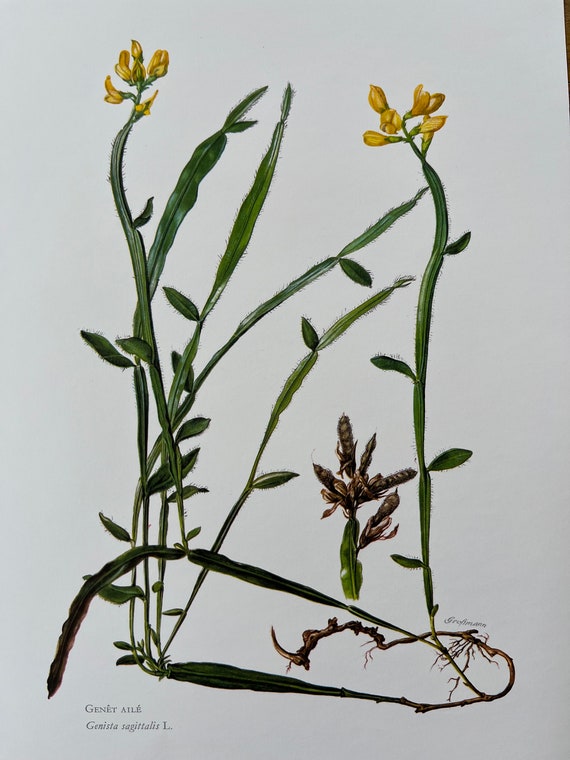The illustration showcases a detailed hand-drawn image of flowers on a pristine white background. Central to the composition are two slender green stalks, slightly offset left and right but predominantly centered. At the top of each stalk, clusters of small, yet-to-bloom yellow buds are visible—five on the left stalk and seven on the right. These delicate buds are complemented by small green leaves lining the stalks. At the base, the roots are clearly depicted, anchoring the plants. A distinct element is a smaller, brownish flower nestled between the two main stalks in the foreground, adding depth to the drawing. Surrounding the primary subjects, some small green blades of grass and additional leaves enhance the naturalistic feel. In the bottom left corner, the artist's name, seemingly "Janay Allay," is inscribed in green writing, providing a personalized touch to this intricate botanical artwork.